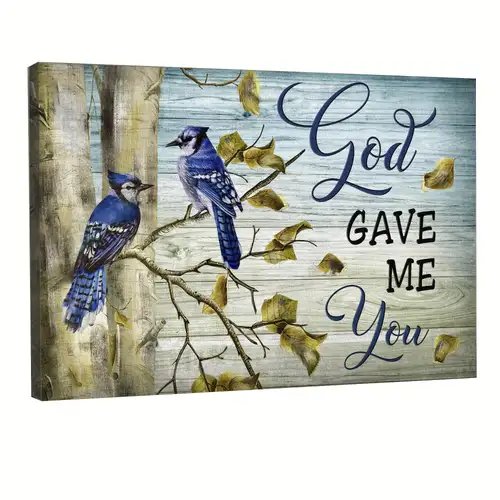The image, intended for wall decoration, displays a serene scene on canvas with a background resembling whitewashed wood that transitions from a bluish tone to light white towards the bottom. On the left side, there are two light-colored birch trees with small, mostly barren branches. Perched on a branch is a blue jay with a triangular head, white around the eyes, and white-sprinkled feathers. On a higher branch, a second blue jay faces the first, distinguished by a slightly darker head and eyes. The leaves on these branches appear dead, with some blowing across the image, enhancing the feeling of a gentle breeze. Inscribed elegantly to the right of the birds are the words, "God gave me you," with "God" and "you" in ornate cursive blue letters, and "gave me" in black block print.